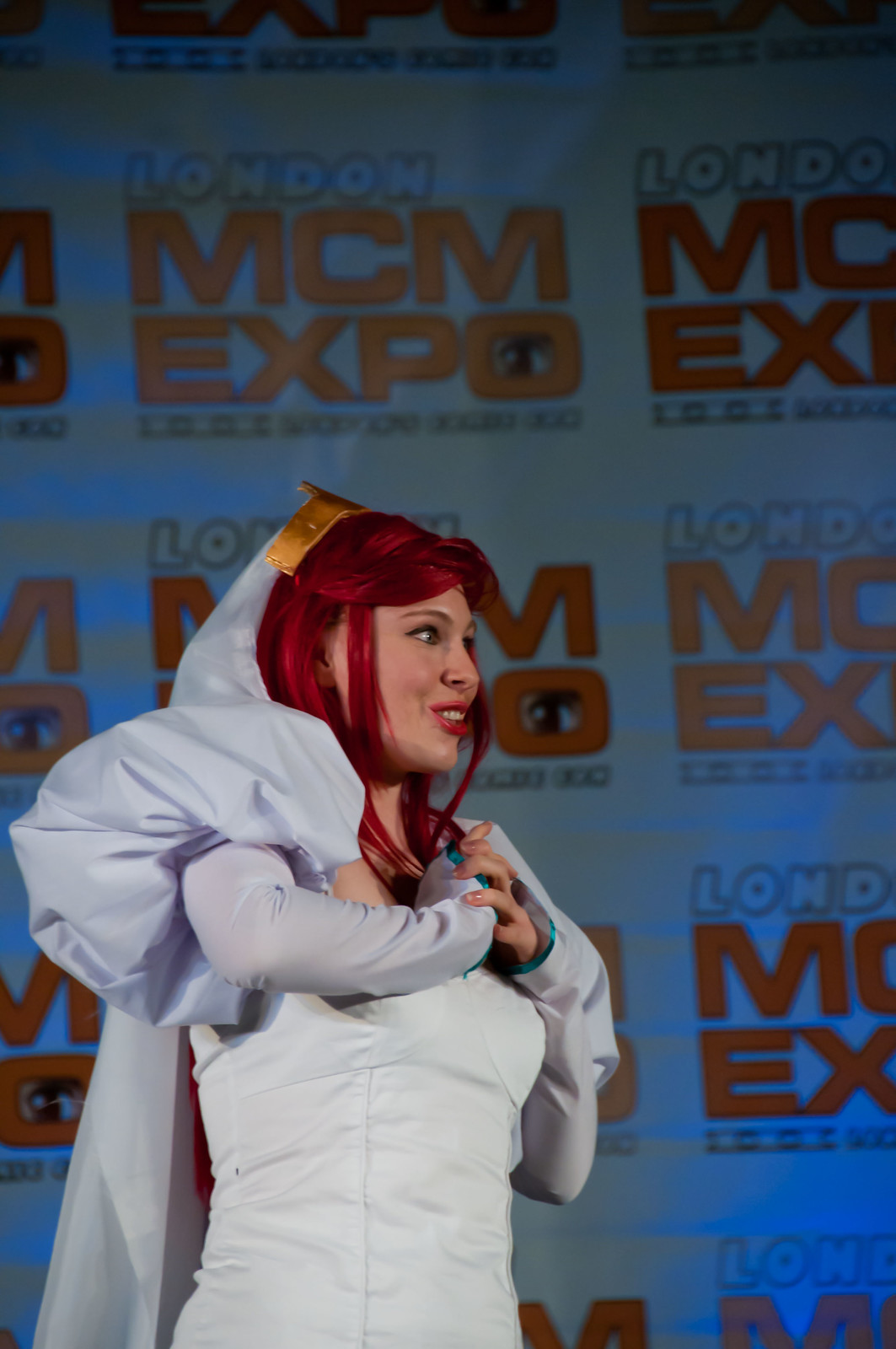The image depicts a woman dressed in an elaborate costume, standing at the center and facing to the right. She has bright red hair, likely a wig, paired with matching bright red lipstick and fair skin. A golden tiara adorns her head, and she wears a smile as her hands are clasped together in front of her chest, making a dramatic gesture. The woman is dressed in a light blue gown with poofy sleeves and a fitted bodice, accentuated by a large, rounded piece of fabric on her shoulder and a long blue cloth draped behind her. The background features a repeating grid pattern of the "London MCM Expo" logo in orange, accompanied by black text, highlighting the event setting.